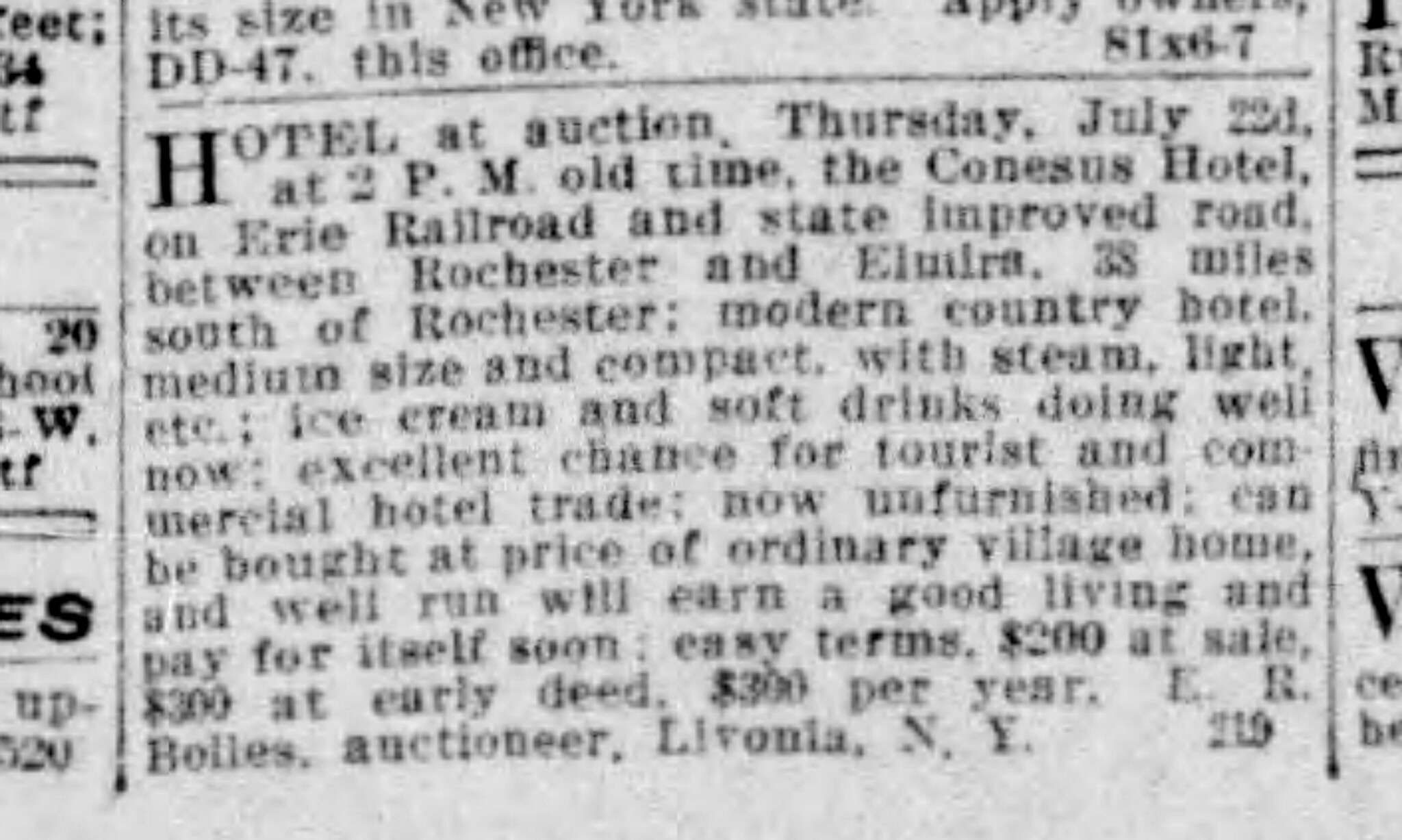This is a close-up photograph of a newspaper clipping that is somewhat blurry, focusing on an auction advertisement for a hotel. The ad, which is in black and white, announces a Hotel at Auction on Thursday, July 22 at 2 p.m. (old time). The specific property is the Canossus Hotel, located on the Erie Railroad and State Improved Road between Rochester and Elmira, 38 miles south of Rochester. The hotel is described as a modern, medium-sized, and compact country hotel with amenities such as steam and light. The advertisement highlights that the hotel currently excels in selling ice cream and soft drinks, presenting an excellent opportunity for both tourist and commercial trade. It is now unfurnished and can be purchased at a price comparable to that of an ordinary village home. The terms are described as easy, requiring $200 at sale, $300 at the early deed, and $300 per year. E.R. Bolas, an auctioneer from Livonia, New York, is handling the sale. There are also some unrelated text fragments on the left and right sides of the clipping, indicating other ads or articles.